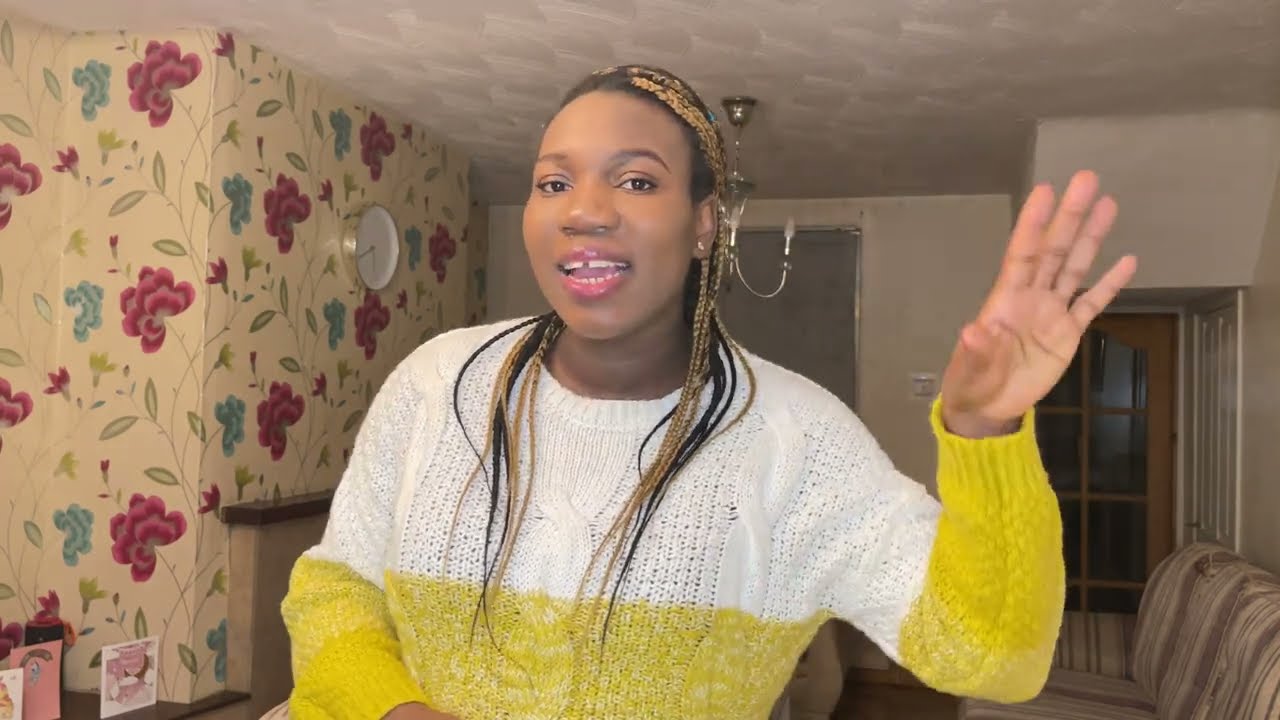The image is a photograph of a woman who appears to be in her living room, visible from the waist up. She is wearing a long-sleeve, cable-knit sweater that is white on the top half and yellow on the bottom half, including the sleeves. She has pink-painted lips and brown skin, her hair styled into long braids that are partially dyed blonde. She is mid-conversation, her mouth open revealing a gap in the front of her upper row of teeth. Her left hand is raised, as if she's emphasizing a point. Behind her, the living room features a ceiling with a pattern, white-painted far-side wall, and a left wall covered with tan floral wallpaper decorated with pink and blue flowers. A gold-rimmed, white-faced clock is mounted on the wallpapered wall. To the right, there's a tan couch with dark tan stripes, positioned against the wall with a glass door or window behind it. On a coffee table in the background are three greeting cards, adding to the homely atmosphere of the scene.